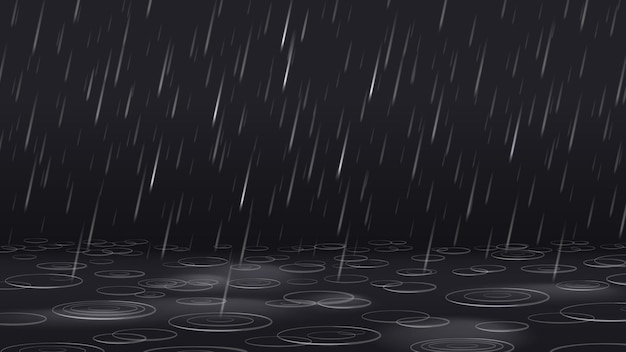This computer-generated image portrays a serene rainfall against a solid black background. White raindrops, resembling streaks or comets, descend at an angle, creating a calming yet somewhat eerie scene. As the raindrops hit the bottom portion of the canvas, they form intricate ripple effects on the surface of a dark pool of water. These ripples overlap, with some displaying multiple concentric circles, adding depth to the simple, monochromatic palette. The absence of any writing or identifiable features, coupled with the stark contrast between the black background and the white raindrops, evokes a sense of quiet solitude, reminiscent of a rainy night illuminated by distant, unseen streetlights.